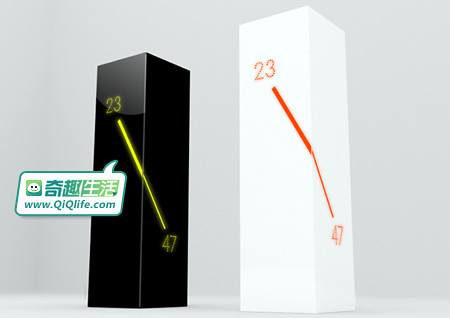This black and white illustration showcases two large 3D rectangular objects set against a grey background with a thin floor at the bottom. The object on the left is black and features a yellow number 23 at the top, a yellow diagonal line descending towards the right, and the number 47 at the bottom. Additionally, there is a speech bubble emerging from this black object, containing a series of small green characters or infographics that are difficult to identify, along with the text "www.qiqlife.com" in green with a white background. The object on the right is white and displays an orange number 23 at the top, a diagonal line descending towards the right and wrapping around the corner, and the number 47 at the bottom. Both objects are slightly angled, facing towards the left.